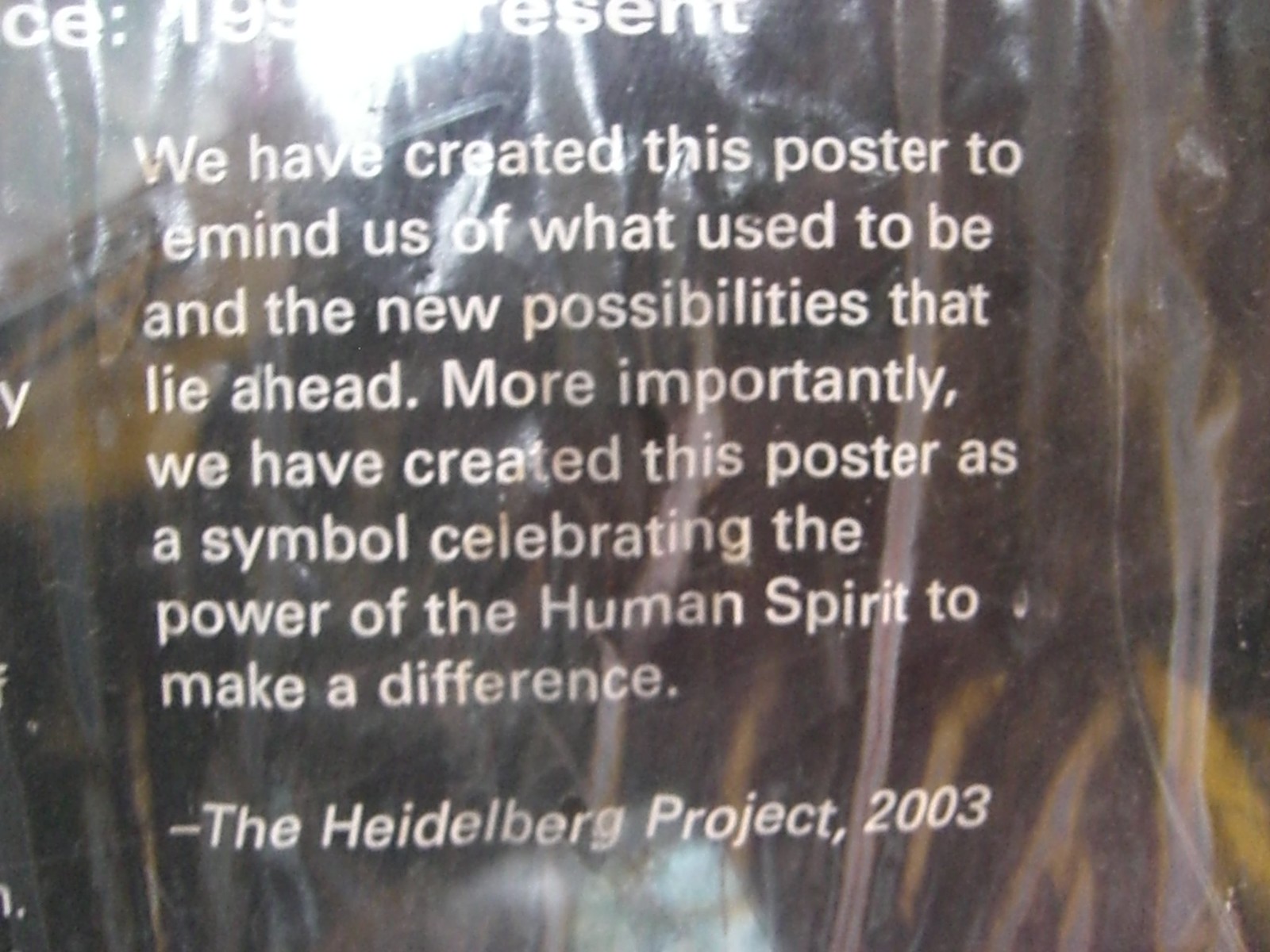The image depicts a reflective, almost see-through, rubbery plastic material, akin to the texture of a raincoat. Despite the zoomed-in nature that makes it difficult to discern the exact object, it features distinct white text centrally positioned in the frame. The text reads, "We have created this poster to remind us of what used to be and the new possibilities that lie ahead. More importantly, we have created this poster as a symbol celebrating the power of the human spirit to make a difference. - The Heidelberg Project, 2003." The background showcases a mix of colors including shades of gray, yellow, tan, black, white, silver, and some hints of red and blue, although the exact nature of these colors remains indistinguishable. The image quality appears somewhat low, adding to the faded, reflective effect seen throughout the scene. This composition suggests the poster might be displayed in a public place, emphasizing the celebration of human resilience and forward-looking optimism.